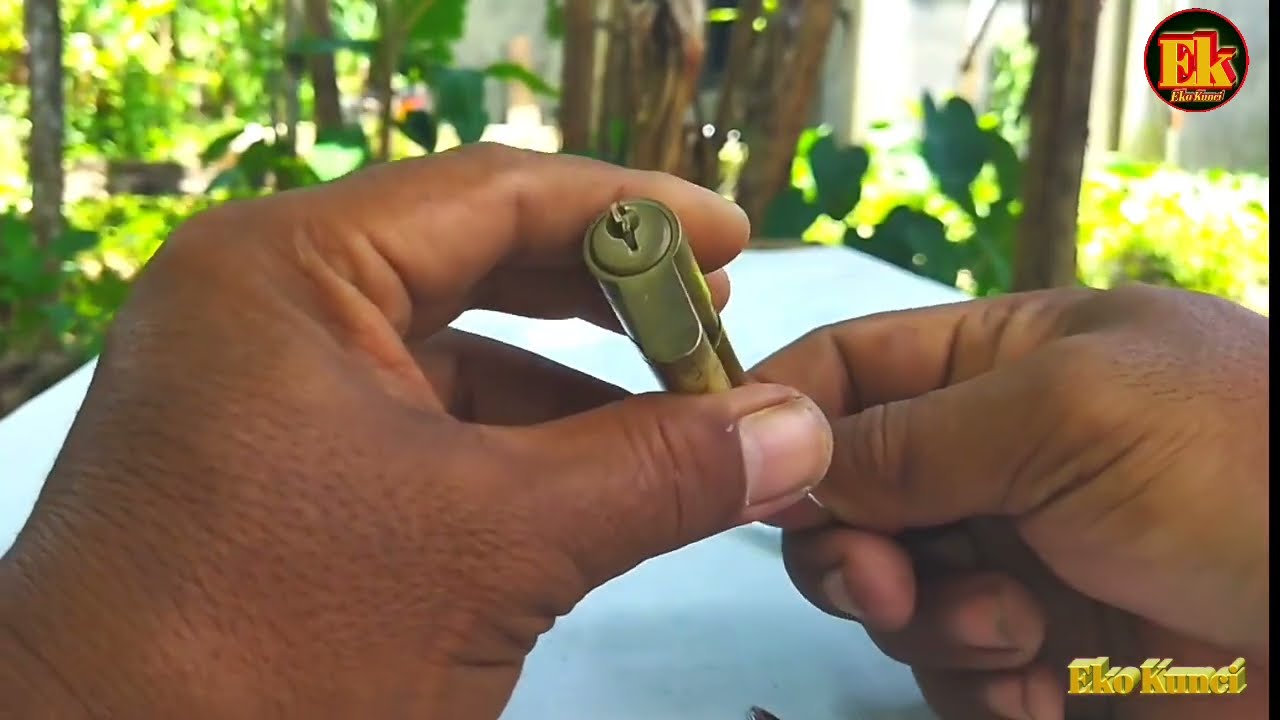The image captures a close-up view of a man's hands, with dark brown skin, holding a brass-like cylindrical object that resembles a lock mechanism with a keyhole on one end. The hands, featuring well-groomed nails, are positioned above a long white table. The background reveals an outdoor setting filled with lush green plants and brown trees, illuminated by bright sunlight. Inscribed in the lower right corner of the image is the text "ECHO KUNCI," while the upper right corner features a yellow circular symbol with the letters "EK."